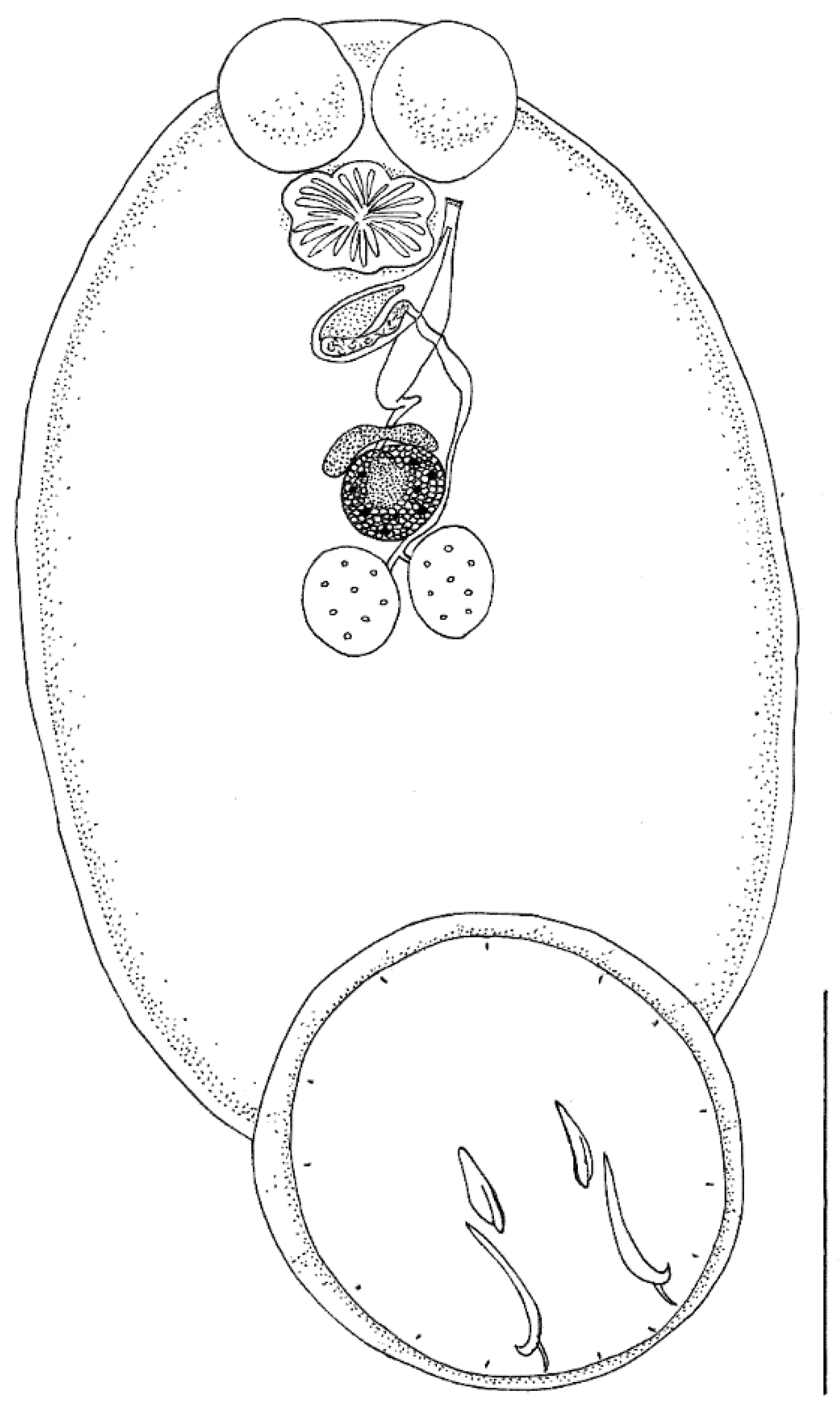The illustration is a detailed black and white drawing featuring an elliptical shape at its center. At the very top of the ellipse are two imperfect circles filled with small black dots, resembling a pair of ovaries or flower petals. Below these are a dark-shaded circle and a shape reminiscent of a lily pad with a flower inside. Further down, more circular objects adorned with polka dots or wisp-like lines emerge; these details evoke the delicate structure of flowers or fruits. At the bottom of the elliptical shape is a larger, circular object with an outer and inner black line border, containing what appears to be string-like elements going through it. An intricate branch or vine-like structure connects these circular forms, adding to the botanical essence of the illustration. The entire composition is framed with delicate brush-like strokes, accentuating its organic and whimsical nature.